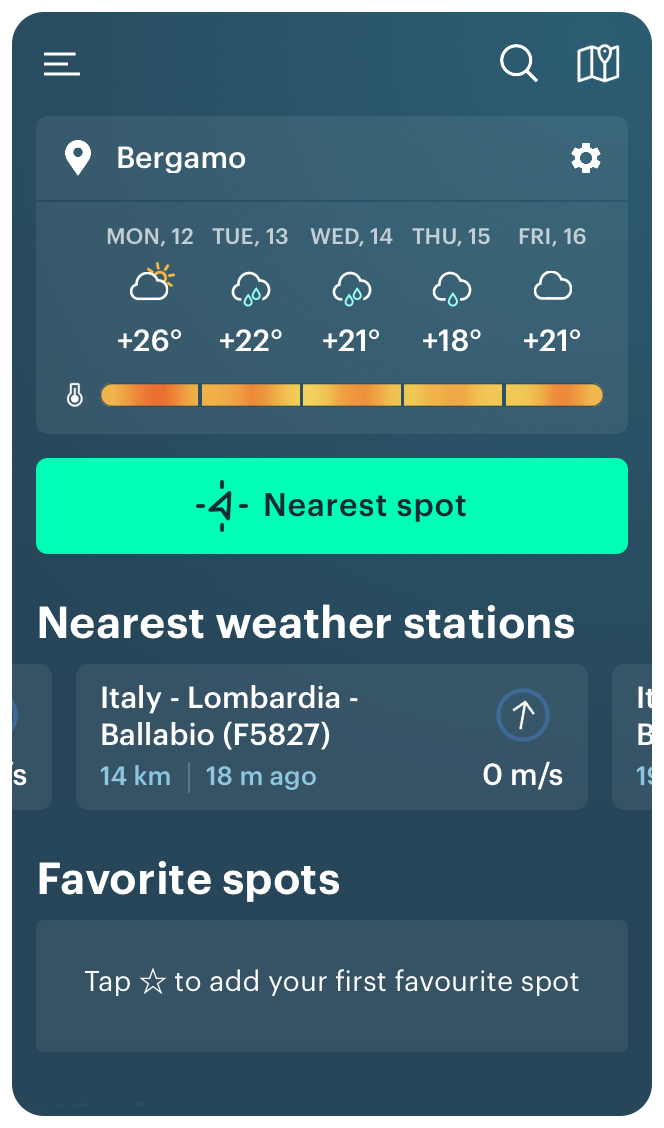This image is a detailed screenshot of a weather app displayed in portrait format, typical for a smartphone screen. The interface features a dark blue background with white text for clear readability. 

In the top left corner, there's a menu icon, and on the top right, there's a search button alongside another icon that resembles a folded map with an upside-down teardrop pointer. 

The weather information is for Bergamo, Italy, covering the week from Monday the 12th to Friday the 16th. Each day's forecast icon indicates varied weather conditions: general cloud cover for all days, with rain on Tuesday, Wednesday, and Thursday, and partly cloudy conditions on another day. Temperatures are displayed in Celsius, supported by a color-coded thermostat bar indicating heat levels, with orange denoting higher temperatures.

Beneath the forecast, there's a green button with black text labeled "Nearest Spot." Further down, the app lists local weather stations in the vicinity of Bergamo, specifically in Italy, Lombardia, and Bellavio, all approximately 14 kilometers away. Users can also save their favorite locations by tapping a star icon.